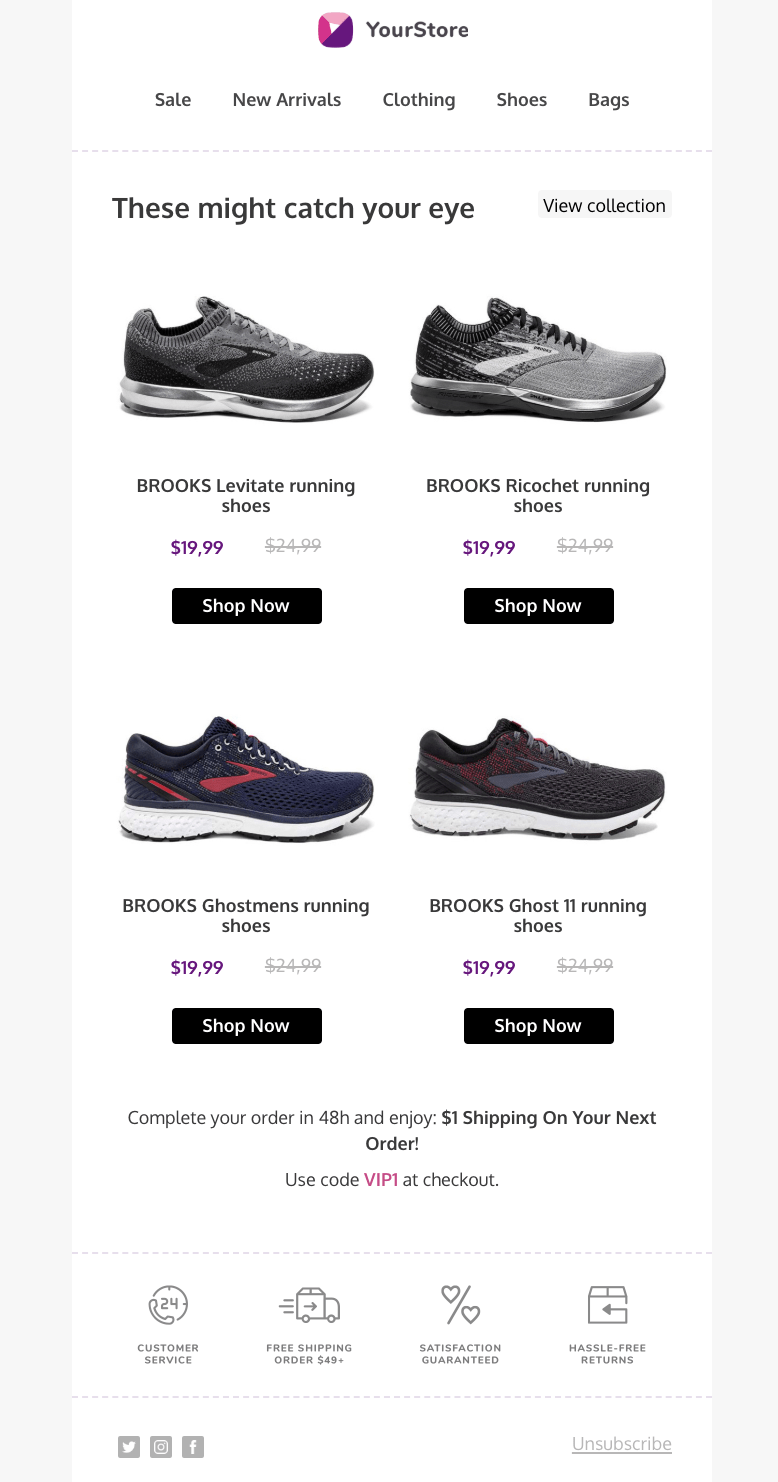The image depicts a store named "Your Store," prominently displayed at the center top of the screen. Below the store's name and logo lies a navigational header listing categories from left to right: Seal, New Arrivals, Clothing, Shoes, and Bags. A dotted line runs horizontally beneath these headings, leading to a bold header titled "These Might Catch Your Eye." To the right of this header is a button labeled "View Collection."

Under this section, a selection of running shoes is showcased, each priced at £19.99, reduced from their original price of £24.99. The shoes featured are:
1. Brooks Levitate Running Shoe
2. Brooks Ricochet Running Shoe
3. Brooks Ghostman Running Shoes
4. Brooks Ghost 11 Running Shoes

Each shoe listing includes a prominent "Shop Now" button in black with white text for easy purchasing. The discounted prices are highlighted in purple, while the original prices are displayed in grey and struck through to indicate the discount.

At the bottom of the screen, four icons represent the store's policies and services: Customer Service, Free Shipping, Satisfaction Guaranteed, and Hassle-Free Returns.